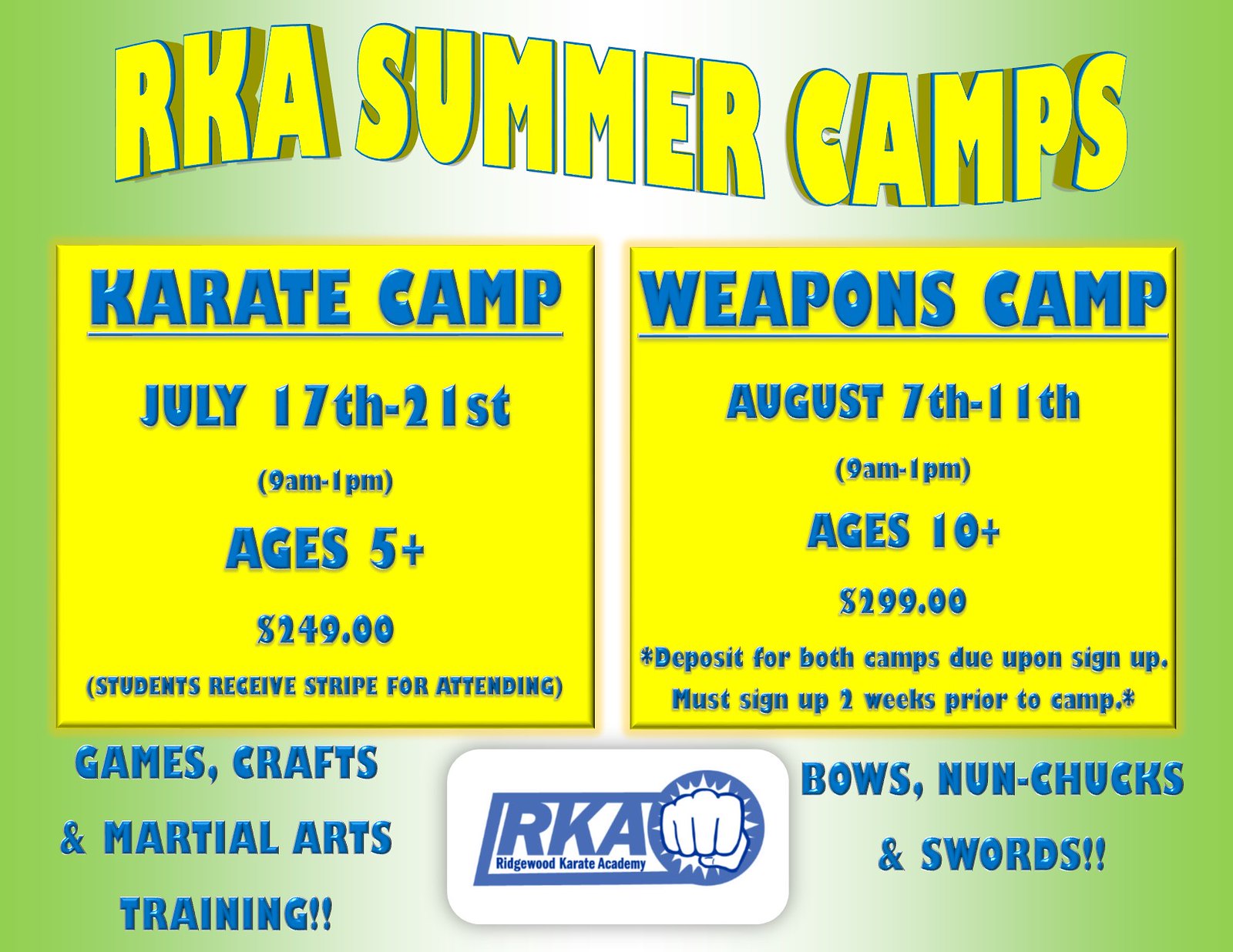The advertisement features a gradient background transitioning from green on the sides to white in the center. At the top, bold, wavy yellow text with a blue outline reads "RKA Summer Camps," casting shadows to the left and right. Below, two yellow squares with blue text detail specific camp information. The left box describes the "Karate Camp" held from July 17th to 21st, 9 a.m. to 1 p.m. for ages 5 and up, costing $249.00, and notes that students receive a stripe for attending. The right box outlines the "Weapons Camp" from August 7th to 11th, 9 a.m. to 1 p.m. for ages 10 and up, costing $299.00, with both camps requiring deposits upon sign-up and registration at least two weeks in advance. Additional text mentions "Games, Crafts, and Martial Arts Training," as well as "Bows, Nunchucks, and Swords." The image also features the logo of RKA Ridgewood Karate Academy, depicting a fist punching forward.